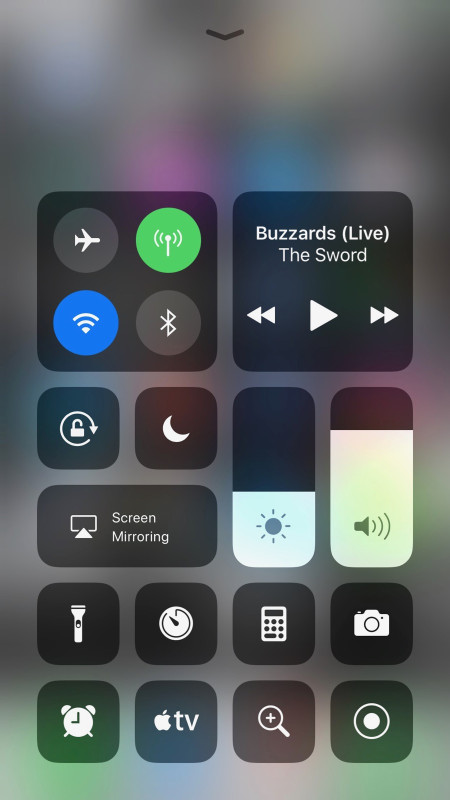The image is a screenshot captured from a cell phone, displaying a blurred background with a focused view of a pop-up menu from a drop-down interface. At the top of the screen, there is a small black arrow pointing downward, indicating the origin of the drop-down menu.

On the menu, arranged in two rows of circular icons:
- The first icon, an airplane, represents Airplane Mode.
- The second icon, a green circle with signal bars, symbolizing cellular signal strength.
- The third icon, on the second row, features a blue background with a Wi-Fi signal indicator.
- The fourth icon depicts a Bluetooth symbol.

To the right of these icons is a square labeled "Buzzards," marked as "live" in parentheses. Below this label are playback controls including a rewind, forward, and play button.

Further down, additional icons are visible:
- A lock icon for screen locking.
- A moon icon, suggesting a Do Not Disturb mode.
- An option labeled "Screen Monitoring."
- Two vertical rectangles with soft edges for adjusting volume and light display.
- Icons for a flashlight, alarm, Apple TV, clock, calculator, camera, search function, and a recording tool.

This detailed and organized layout of the menu provides quick access to essential phone features and settings.